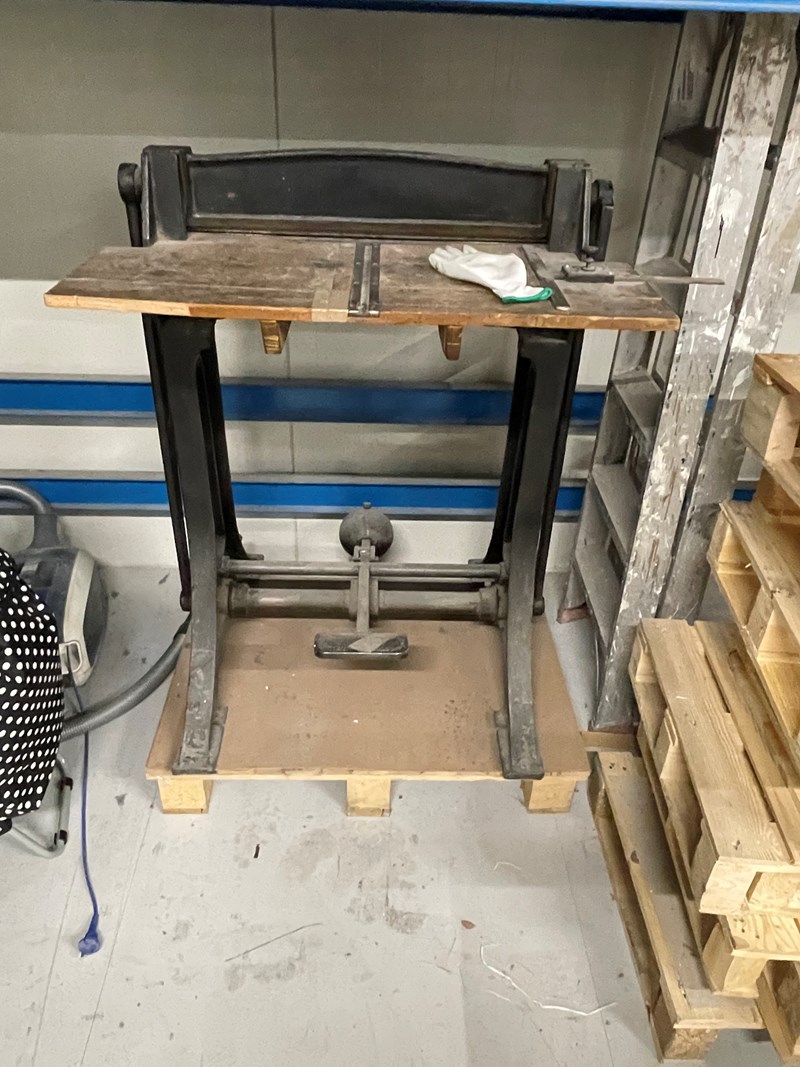This photograph captures a vertically aligned, rectangular image of a vintage woodworking vise situated in a semi-industrial workshop, possibly a woodworking or artistic environment. Central to the composition is a wooden stand with a heavy black steel frame featuring four robust feet. The vise appears integrated into the wooden tabletop, which is about three feet wide, and is operated by two black twist pieces and a pedal mechanism at its base. 

Atop the wooden surface lies a white work glove and some scattered white dust. Adjacent to the vise, on the lower left, rests a black and white polka dot bag. To the right are stacks of wooden pallets, divided into rectangular sections.

The background consists of white wall panels accentuated by blue horizontal stripes running parallel across the lower section. The floor seems to be constructed of white tiles, littered with edges of wooden crates, contributing to the workshop's somewhat cluttered appearance. Evident in the scene are various objects including a narrow gray shelf marked with stray brush strokes, a cord trailing towards the front, and what might be a vacuum cleaner with a polka-dotted bag.